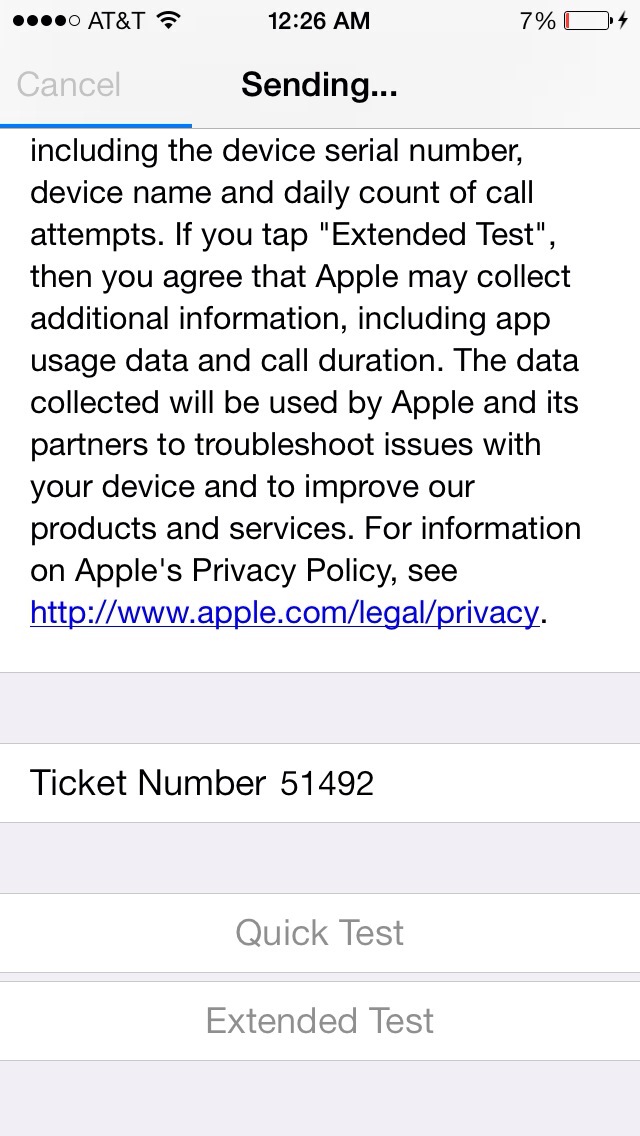The image is a screenshot of an AT&T iPhone screen displaying a partially sent message. At the top left corner are five circles, four filled and one clear, followed by "AT&T." Next to that, a fully filled Wi-Fi signal symbol is visible, and the time in the center reads 12:26 AM. On the right side, the battery icon shows 7% remaining with a small red bar, indicating it is almost out of power. 

Below this status bar, the message status is displayed with a grayed-out "Cancel" button on the left and "Sending..." with a blue progress bar that is about one-third complete. Below this, there is an extract of an email message detailing that if the user taps "Extend Test," they agree to allow Apple to collect additional information such as app usage data and call duration to troubleshoot device issues and improve services. A privacy policy link is provided: http://www.apple.com/legal/privacy.

Further down, "Ticket number 51492" is shown, followed by two grayed-out buttons labeled "Quick Test" and "Extended Test." The screen ends with another small gray bar at the bottom.